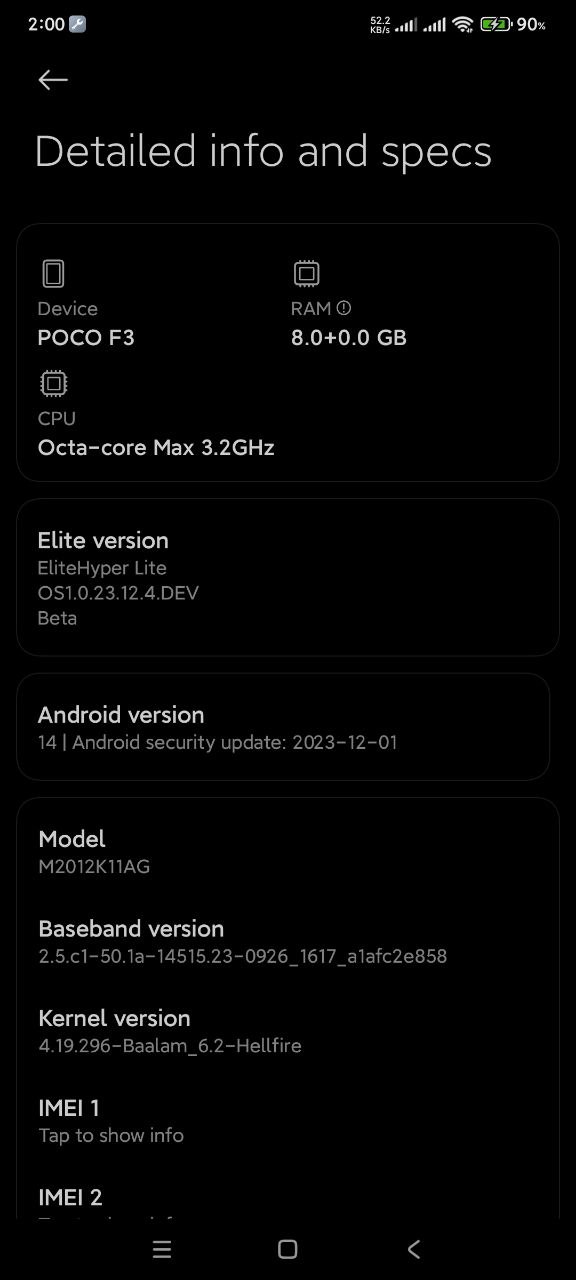A detailed screenshot of a smartphone display features a black background. At the top left, a timestamp reads "2:00". Adjacent to the time, there's a wrench icon, followed by a Wi-Fi symbol, and a battery icon showing 90% charge.

Beneath this top row, a left-facing arrow is visible, below which the text "Detailed Info and Specs" appears, indicating information about either the smartphone itself or its operating system.

In the central section of the screenshot, there's an image of a device labeled "Device - POCO F3". To the right of this image, a card is displayed showing "RAM: 8.0 + 0.0 GB". Directly below, another card presents details about the CPU: "Octa-core max 3.2 GHz". 

Further down, the text "Elite Version: Elite Hyperlite OS 1.0.23.12.4.DEV BETA" is shown, followed by "Android Version: 14 - Android Security Update: 23-12-01". Beneath this, information about the model is listed as "Model: M2012K11AG". 

Additional specifics include the baseband version "2.1C1-50.18-14515.23-0926_1617_A1AFC2E858" and the kernel version, followed by two identifications labeled "IMI1" and "IMI2".

Finally, at the bottom of the screenshot, standard navigation icons are displayed: a hamburger menu, a home button, and a left-facing arrow.